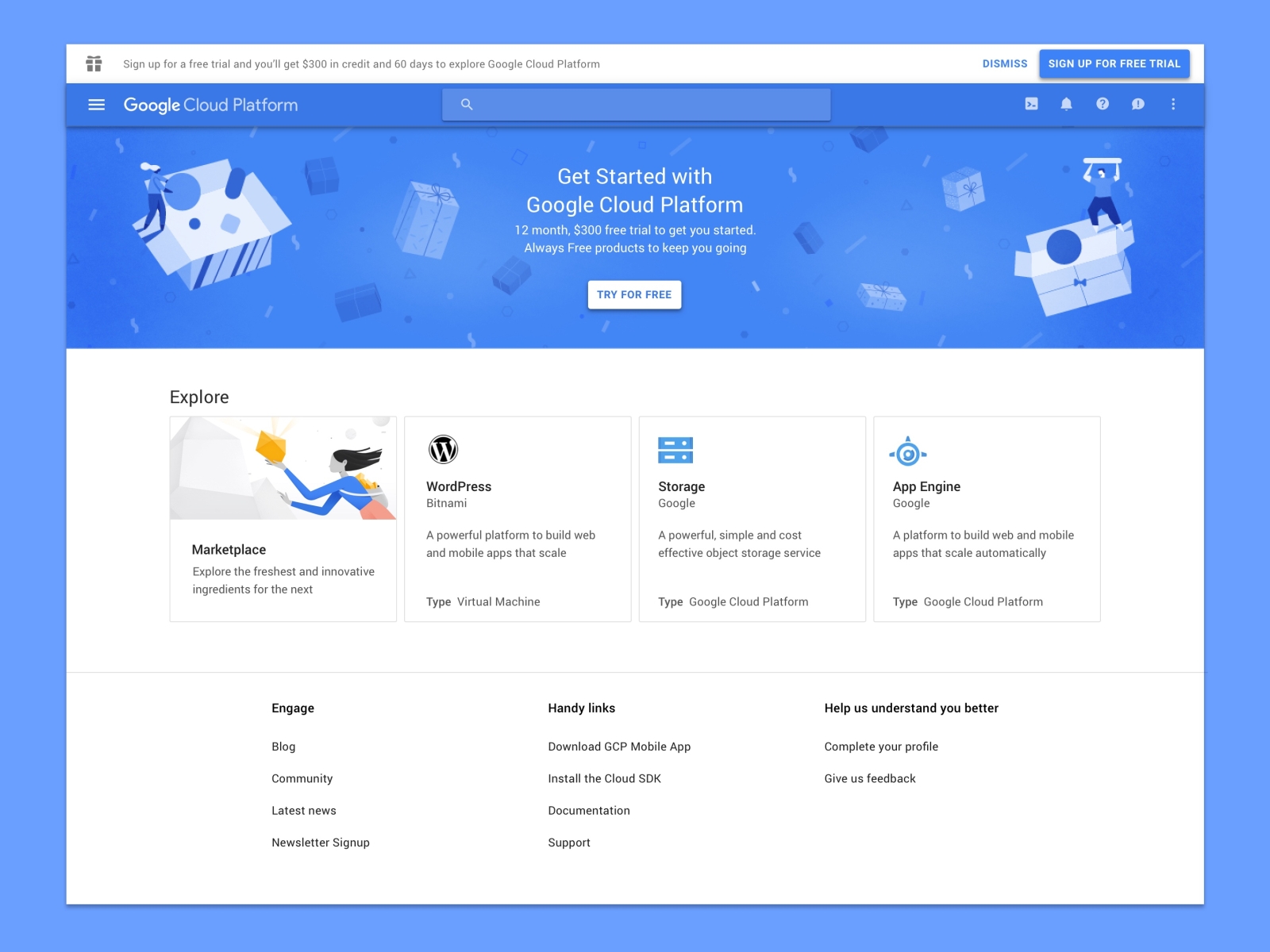Screenshot Description:

The presented image features a baby blue border encompassing the entire screenshot. At the top of the image, there is a white horizontal bar accompanied by a very dark blue present icon on the left side. Just below this, blue text reads: "Sign up for a free trial and get $300 in credit. 60 days to explore Google Cloud Platform." Following this text is a white space, with a white "Dismiss" button situated on the right side.

Continuing downward, there is another area with a blue dominant color. In white text surrounded by blue, it reads: "Sign up for a free trial." Below this text, additional blue elements are present, and "Google Platform" is inscribed in white. A blue search icon, followed by various other icons including a calendar, a bell, a question mark, an exclamation point, and three dots, are also visible.

Below these elements is another blue section featuring two presents being opened, illustrated in varying shades of blue with people depicted as standing in them and extracting contents. At the center, white text states: "Get started with Google Cloud Platform. 12-month $300 free trial. Always free products to keep you going." Beneath this message, a prominent blue button with white text reads: "Try for free."

The lower portion of the image is dominated by a large white area filled with black text detailing various features such as Marketplace, WordPress, Storage, and App Engine. This section includes extended information alongside multiple button links for further actions and exploration.